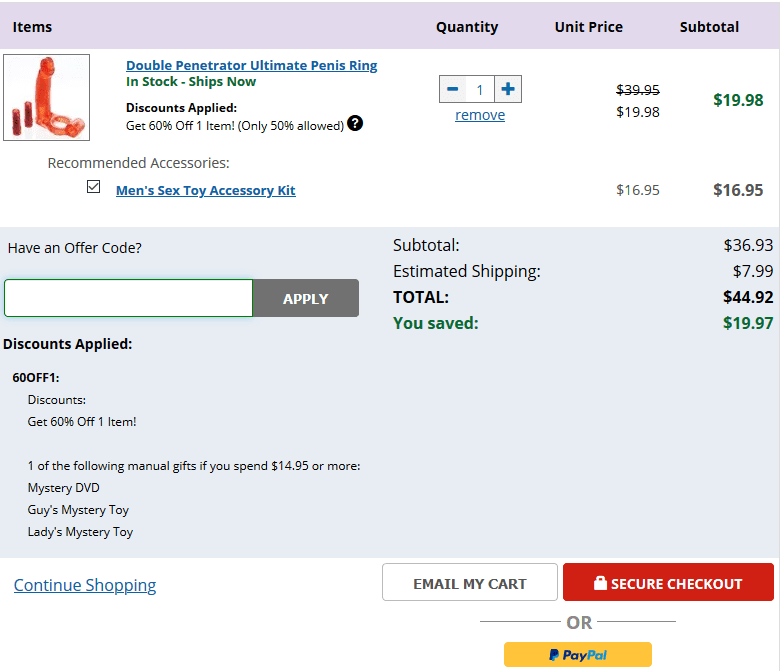The image captures a transaction page featuring a detailed list of items for sale against a subtle, light purple background. At the top of the page, headings such as "Items," "Quantity," "Unit Price," and "Subtotal" are displayed in black text. 

Beneath these headings, an image prominently features a product labeled "Double Penetrator Ultimate Penis Ring." To the right of the image, the product name is highlighted in blue. In a muted green font below the product name, it states "In Stock – Ships Now." Further down in black text, there's a bold proclamation "Discount Applied." Following this, an attention-grabbing note in black reads, "Only 50% off one item! Only 50% allowed!" accompanied by a question mark inside a circle.

Additionally, a rectangular box displays the quantity of the item as "1," flanked by a minus sign on the left and a plus sign on the right to adjust the quantity. Under the "Unit Price" section, the original price of $39.95 is struck through, revealing a discounted price of $19.98. Correspondingly, under the "Subtotal" column, the total price is highlighted in green as $19.98, confirming the applied discount.